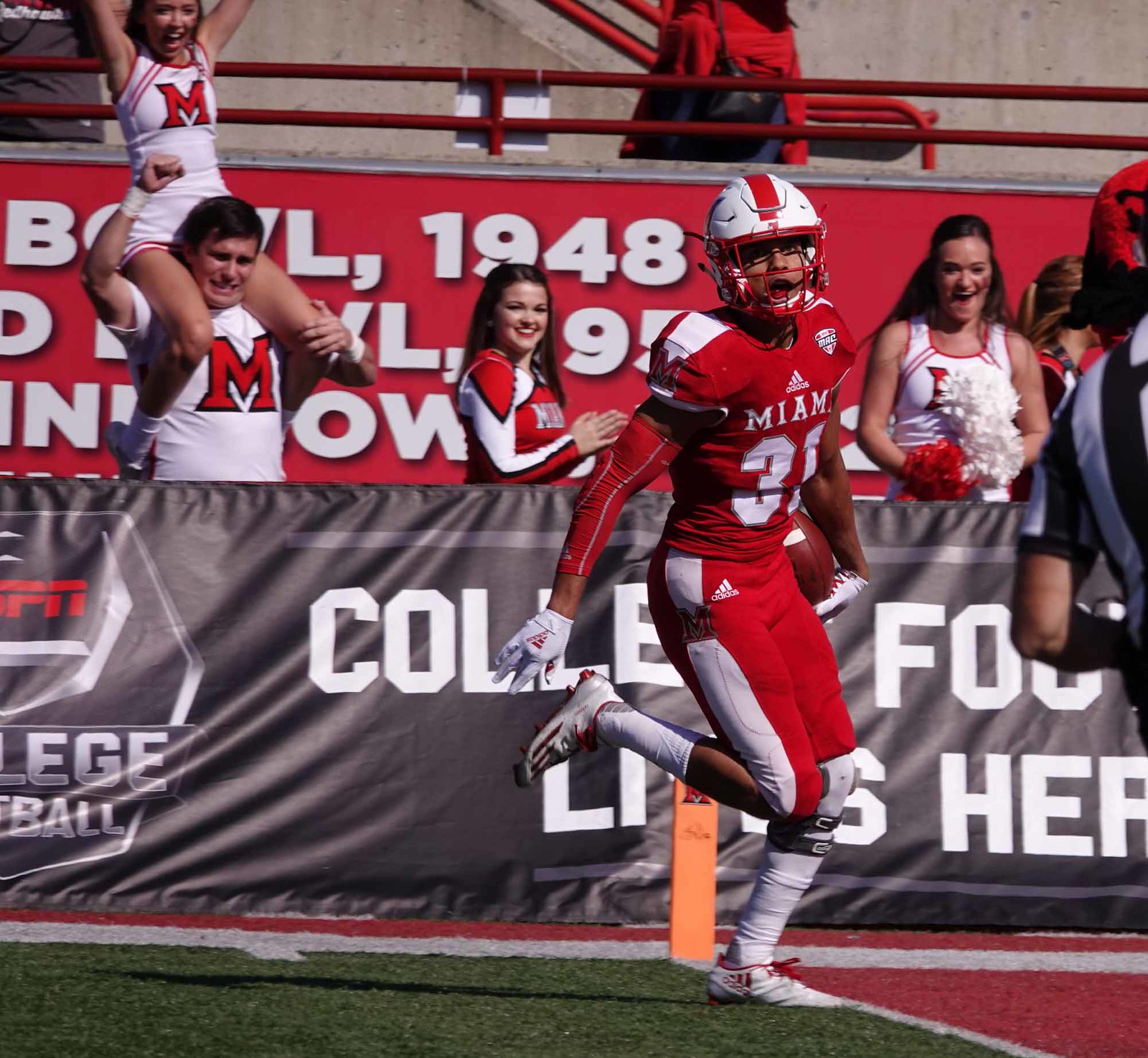This detailed photo captures an exhilarating moment in a college football game. At the center, a Miami football player, clad in a red and white uniform with a helmet featuring red stripes, has just reached the touchdown line. He holds the football in one arm by his side, with one knee up and the other leg slightly bent, mouth slightly open as if caught in motion. Positioned right at the goal line, identifiable by the white lines and the orange cone marking the touchdown area, he celebrates his triumphant run. In the vibrant background, a sunny day highlights a scene full of excitement: cheerleaders, also in red and white, cheer enthusiastically. One cheerleader perched on another's shoulders stands out, while others wave pom-poms and clap joyfully. A prominent black banner with large white letters declares "College Football Lives Here," and an ESPN logo further emphasizes the collegiate atmosphere of this thrilling game.